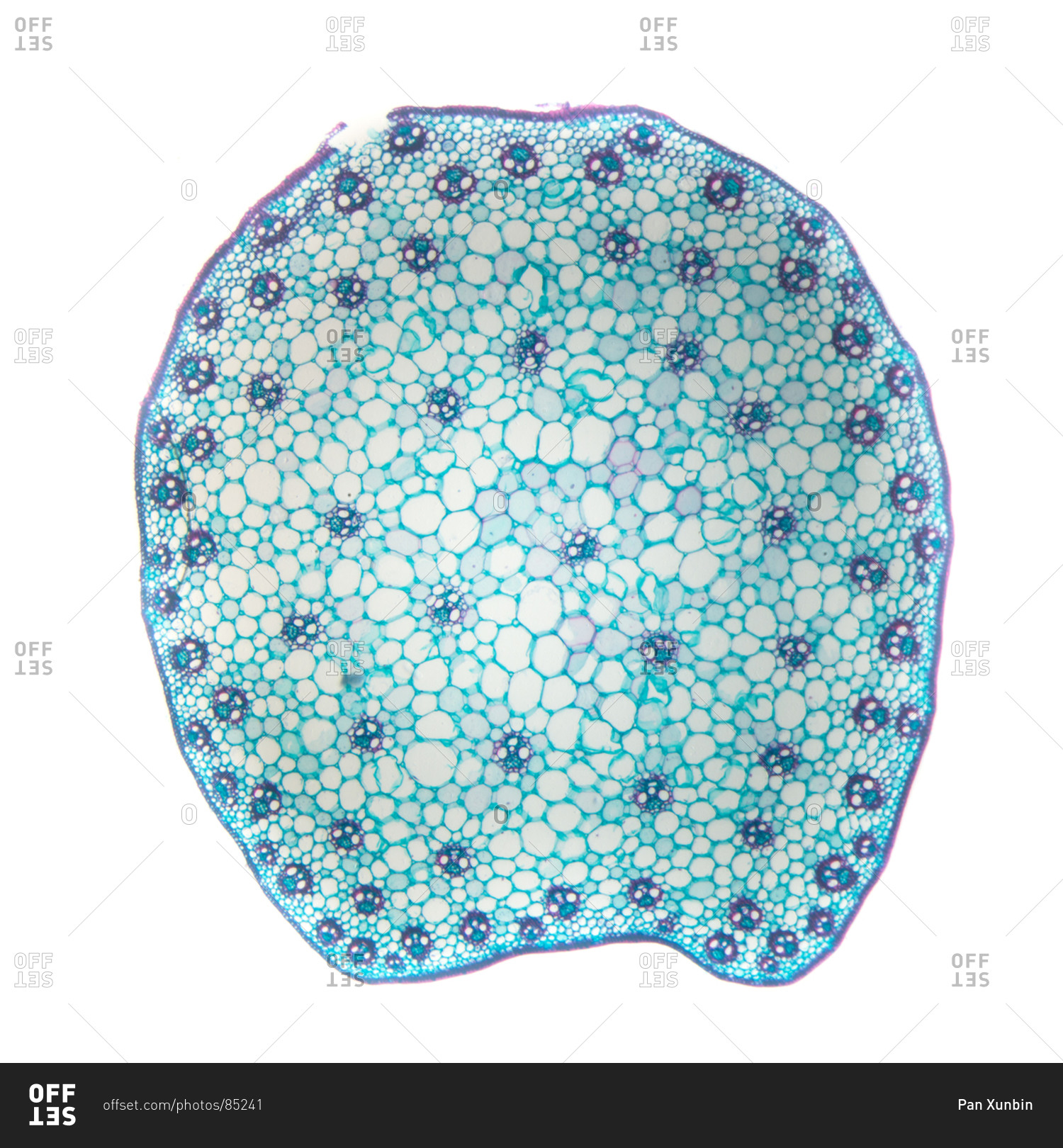This illustration features a close-up, detailed depiction of a microscopic cell slice. The irregular, rounded cell is predominantly light blue with a dark blue outline. Inside, it is segmented into various smaller, irregular circular shapes that give the appearance of cells-within-cells. These smaller cells are primarily white with a blue aqua background. Scattered throughout the cell are darker blue circular segments, creating a bubble-like texture, with a higher concentration near the edges. These darker segments are composed of even smaller shapes, mixing white, blue, and dark blue colors. The image is watermarked with gray text that says "OFF" on top of "SET," the latter being upside down, repeated multiple times across the cell. A dark gray bar at the very bottom carries the branding and contact information, reading "offset.com/photos/85241" on the left and "Panzunbin XUNBIN" on the right.